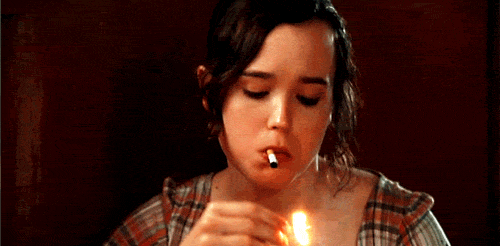In this short movie clip, a young Caucasian woman, possibly a TV star, is lighting a cigarette. She is viewed from the shoulders up against a dark backdrop that shifts from black to a deep, rust brown hue as the flame flickers. She appears to be between 18 and 20 years old, with dark brunette hair slightly pulled back, leaving a few tendrils framing her face. Her dark eyebrows and eyelashes accentuate her features. Wearing a plaid top with a low V-neck that exposes her shoulders, she uses her right hand to strike a match and light the cigarette held in her mouth. The scene focuses on this repetitive action of lighting the cigarette, emphasizing the contrast between the bright match flame and the dark, reddish-brown background. The clip captures a moment of raw, quiet intimacy.